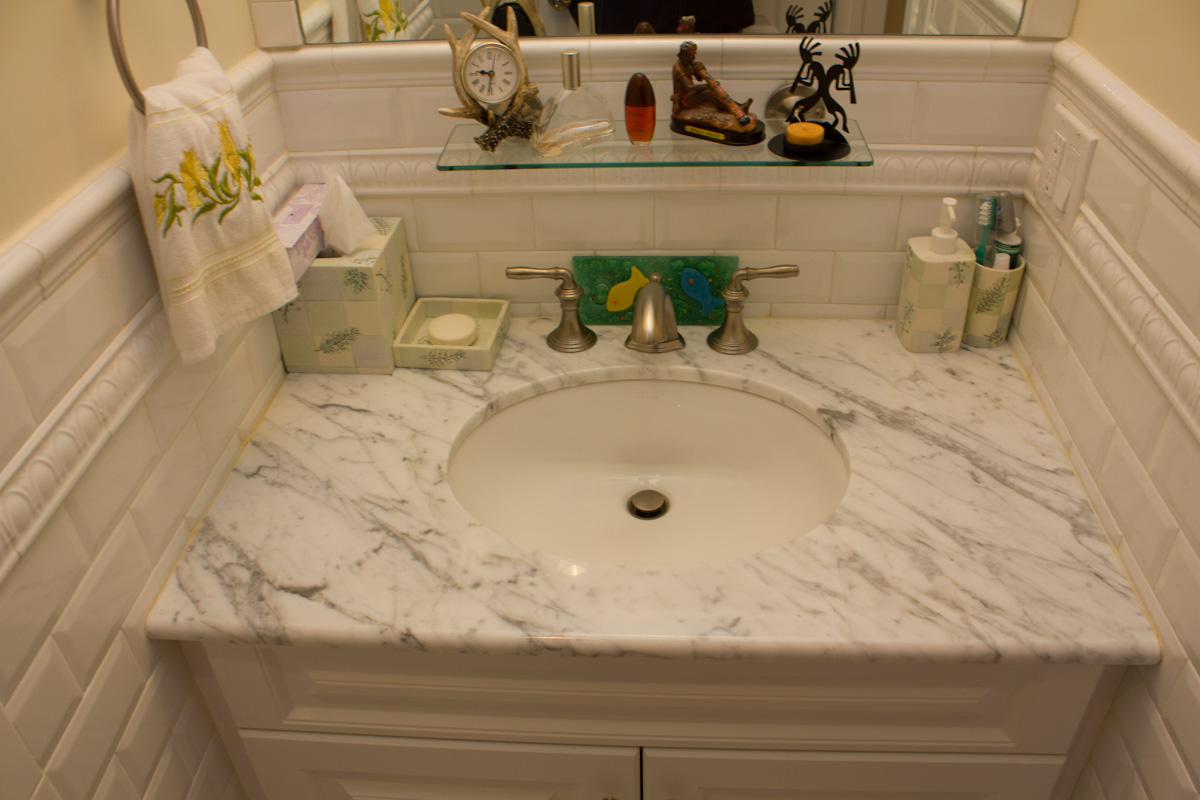The image showcases a bathroom corner focusing on a meticulously arranged countertop. The countertop, crafted from sleek white and grey marble, is bordered by two walls on either side, making it appear nestled in a corner. Below the marble surface are pristine white drawers providing storage. To the left, a ring holds a vivid yellow towel adorned with a cheerful tulip pattern. Above the counter, a white glass shelf is affixed to the wall, displaying an assortment of items including a small clock, various nail polishes, and several decorative pieces among which a miniature sculpture stands out. 

Centrally positioned behind the bronze-colored faucet with matching handles, there is a decorative tablet featuring a fish pattern, adding a whimsical aquatic touch. The soap and toothbrush holder, adorned in a coordinated design, are slightly visible in the reflection of a nearby mirror, though the focus remains primarily on the countertop area itself. The walls of the bathroom are painted in a soft, pale yellow hue, complimented by sections of decorative brickwork that infuse the space with a rustic charm.